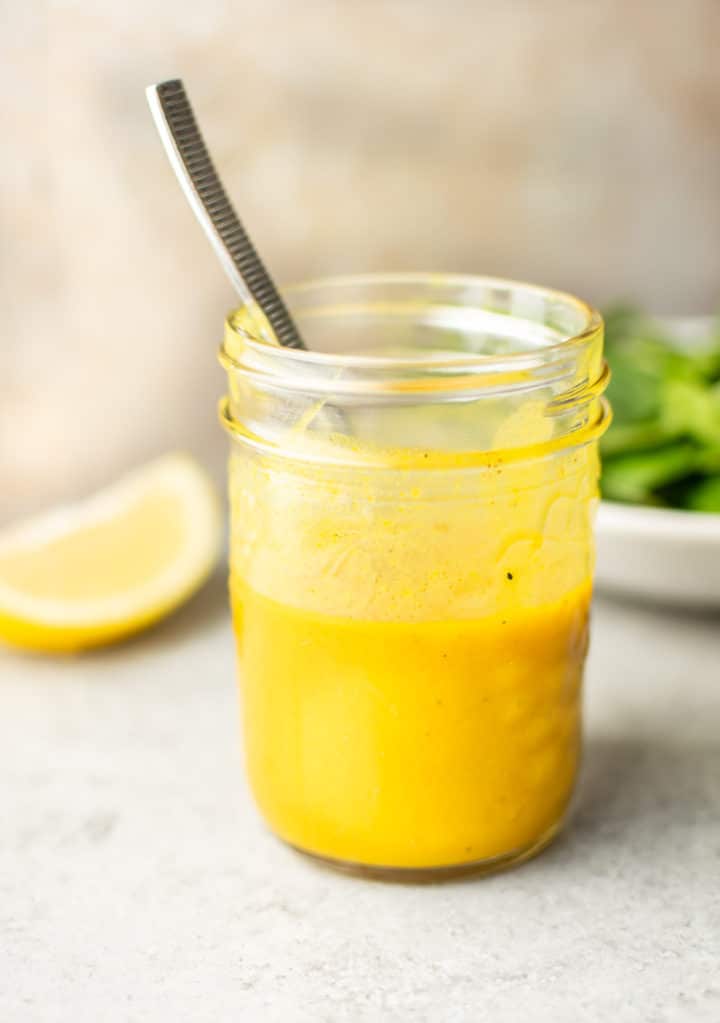This portrait-mode photograph showcases a glass jar centrally placed on a cream-colored marble countertop with a blurry cream background. The jar, which is open and rimmed at the top, contains a thick, vibrant yellow liquid that reaches about halfway up. Emerging from the jar is a silver utensil, possibly a spoon, adorned with striped designs. To the left of the jar lies a slice of lemon, while to the right is a white plate holding green vegetables. The overall scene is serene and minimalistic, capturing the essence of the contents and their relationship with the surrounding items.